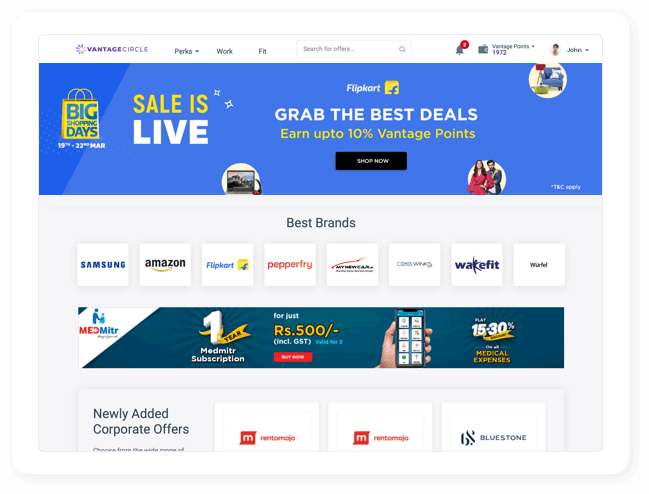**Caption:**

On a sleek white and light blue background, this promotional image is headlined by the "Vantage Circle" logo in blue, adorned with a semi-circle and pointed design. At the top, it features tabs for "Perks" with a dropdown arrow, "Work" and "Fit", alongside a search box, a notification bell with a red circle indicating seven notifications, and the user's Vantage Points total of 1,972. The user profile section shows a thumbnail image labeled "John" with a dropdown arrow.

Dominating the center is a large black box highlighting a promotional event. A yellow grocery bag with the text "Big Shopping Day" in blue announces a sale from March 19th to 22nd. Above, two stars catch the eye, while below, it notes "Sale Live" in white and yellow text, featuring a Flipkart logo inside a yellow square with a blue 'F' symbol. 

In the bottom right corner, a circular white bubble showcases a cozy setup with a blue chair, a blue and white pillow, a yellow pot, and a red lamp, with the text "Grab the best deals" in white and "earn up to 10% Vantage Points" in yellow. Underneath, a black "Shop Now" button prompts action.

Additional promotions highlight a medley of top brands like Samsung, Amazon, Flipkart, Pepperfry, My New, Winks, Wakefit, and Würfel, organized neatly in squares. A side promotion in a white corner with a blue tip showcases "Med Mitzer", with "Med" in red and "Mitzer" in blue, alongside an icon of an adult figure holding a child. 

Further down, a blue promotional box details a "One Year" subscription offer, featuring a white "1" and a yellow ribbon marked "year". The deal offers a "Mad Meter subscription for just RS.500" in bold yellow, including GST, valid for two people, with a prominent red "Buy Now" button. Adjacent, a graphic of a person holding a phone states "Play 15-30%" with a yellow flag underneath, promoting discounts on medical expenses.

The bottom segment showcases newly added corporate offices against a white background, listing "M", "Rent-A-Mojo", "Rent-A-Mojo", and "Bluestone". The image encapsulates a comprehensive promotional campaign with detailed visual and textual elements, designed to attract and inform users.